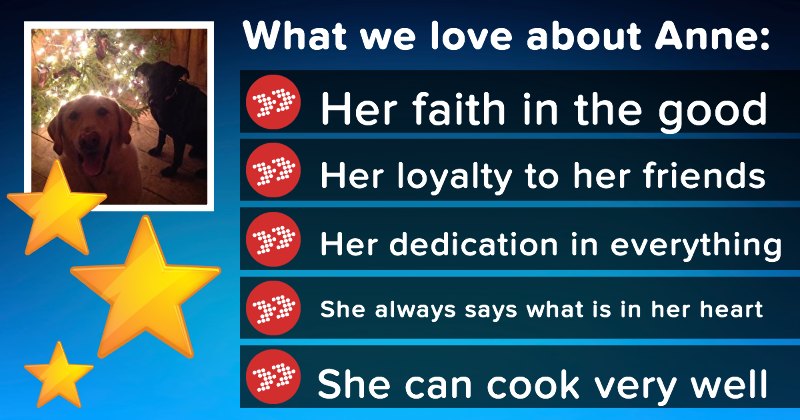This image is a poster that appears to be either from an animal shelter or a tribute to someone named Anne. On the left-hand side, there is an upper section containing a small picture of two dogs—one black and one beige—standing in front of a lidded Christmas tree adorned with white lights. Both dogs are looking at the camera, adding a touch of cuteness to the image. Beneath the picture of the dogs, there are three gold clipart stars—arranged as one on the left, one on the right, and one more on the left. 

The right-hand two-thirds of the poster includes a title that reads "What We Love About Anne:" followed by a list of five attributes, each introduced by red blocks. These points highlight Anne's admirable qualities:
1. Her faith in the good.
2. Her loyalty to her friends.
3. Her dedication in everything.
4. She always says what is in her heart.
5. She can cook very well.

The sign functions as a heartfelt recognition of Anne, possibly indicating her relationship with the dogs or her involvement in the context of the poster.